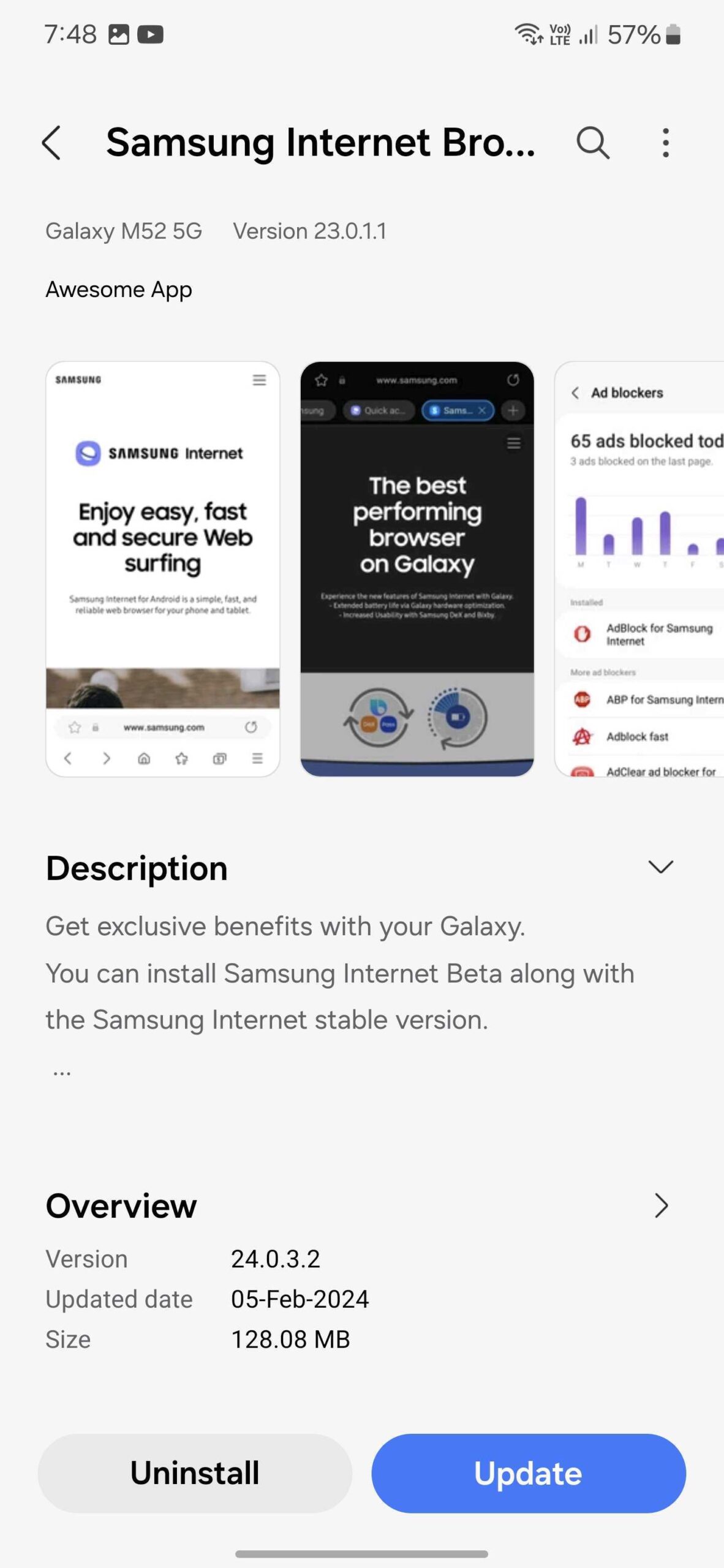The image is a detailed screenshot of a smartphone screen, which is approximately three times taller than it is wide. The background is light gray and features black text throughout. 

In the top left corner of the screen, the time is displayed as 7:48, and in the top right corner, various signal strength icons are visible alongside a battery icon that shows 57% remaining. 

The primary content begins with a left arrow indicating previous navigation, followed by the text "Samsung Internet," a search icon represented by a magnifying glass, and a menu icon featuring three vertical dots. 

Below this, in smaller text on the left side, the screen indicates "Galaxy M52 5G version 23.0.1.1." Directly underneath, bolded text reads "Sync on Black Awesome App."

The main body of the screen features three horizontal ads for the Samsung Internet browser, which can be scrolled through. The ads are: 
1. "Samsung Internet - Enjoy easy, fast, secure web surfing."
2. "Best performing browser on Galaxy."
3. "65 ads blocked today," shown with an accompanying bar graph.

At the bottom of the screen, a section titled "Description" appears, followed by three lines of descriptive text.